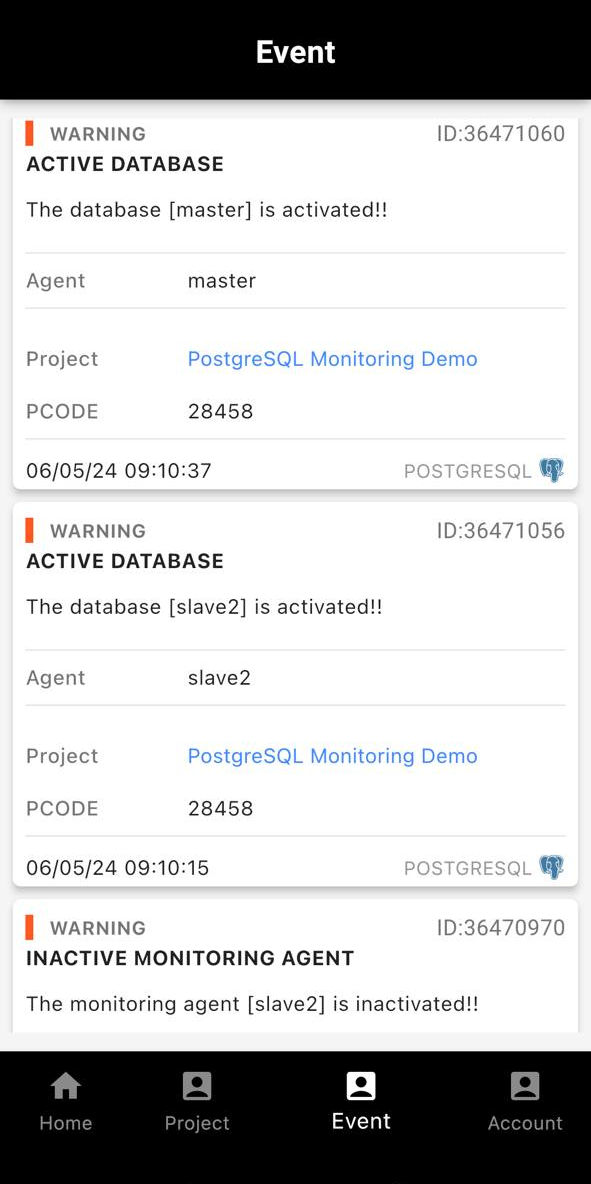This image, captured from a cell phone screen, displays a notification from the "WHATAP service" application. At the top of the screen, a black rectangle prominently features the app’s name in white text: "WHATAP service." Below this, a white speech bubble with an exclamation point inside appears.

In the main white section of the screen, a vertical red line highlights a warning message. The message reads: "WARNING: HITMAP_FLOOD_PATTERN. FLOOD PATTERN WAS DETECTED IN THE PROJECT HITMAP." Below this, additional information is provided: "CODE: 5490, PROJECT: JAVA APM DEMO, AGENT: [agent details], DATE: 12-15-23, TIME: 12:47:00."

Toward the bottom right corner of the screen, an emblematic symbol accompanies the word "JAVA."

Further down the screen are two additional warning messages, similar to the first. The second warning is timestamped "12:36:00," and the third appears with the time "12:26:00." Each message indicates ongoing issues detected in the HITMAP project at various intervals.